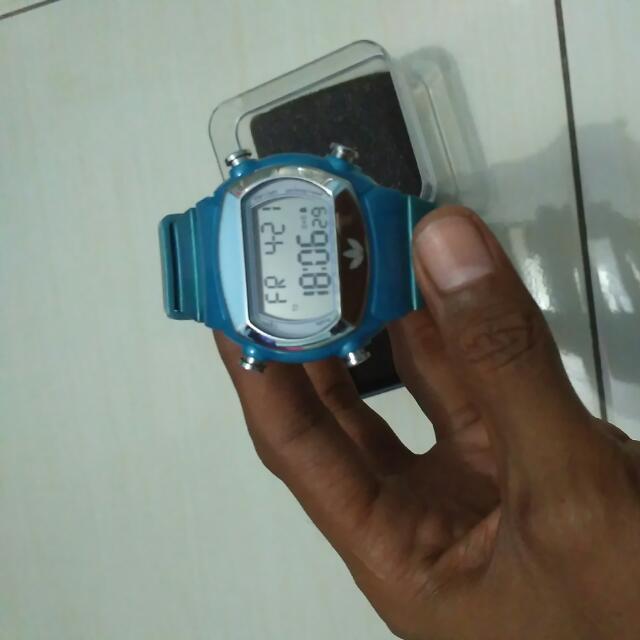A detailed image shows a dark-skinned left hand, likely of an African-American, emerging from the lower right corner of the frame, with pinkish nails visible on the thumb. This hand is holding a blue digital wristwatch between the thumb, forefinger, and middle finger. The watch is presented sideways, positioned horizontally in the center of the picture, and displays "FR 4-21" and "18:06:29" on its light gray face with dark gray or black numbers. Below the screen, there appears to be a logo resembling the Adidas three-leaf symbol. The background is a solid light gray, suggesting a plain door or a light-colored table as the setting. The wristwatch features four silver buttons, two on each side, and casts a shadow to the right. It has just been taken out of a clear square plastic container with a black insert, which is situated above the watch, indicating it was previously on a glossy white surface.